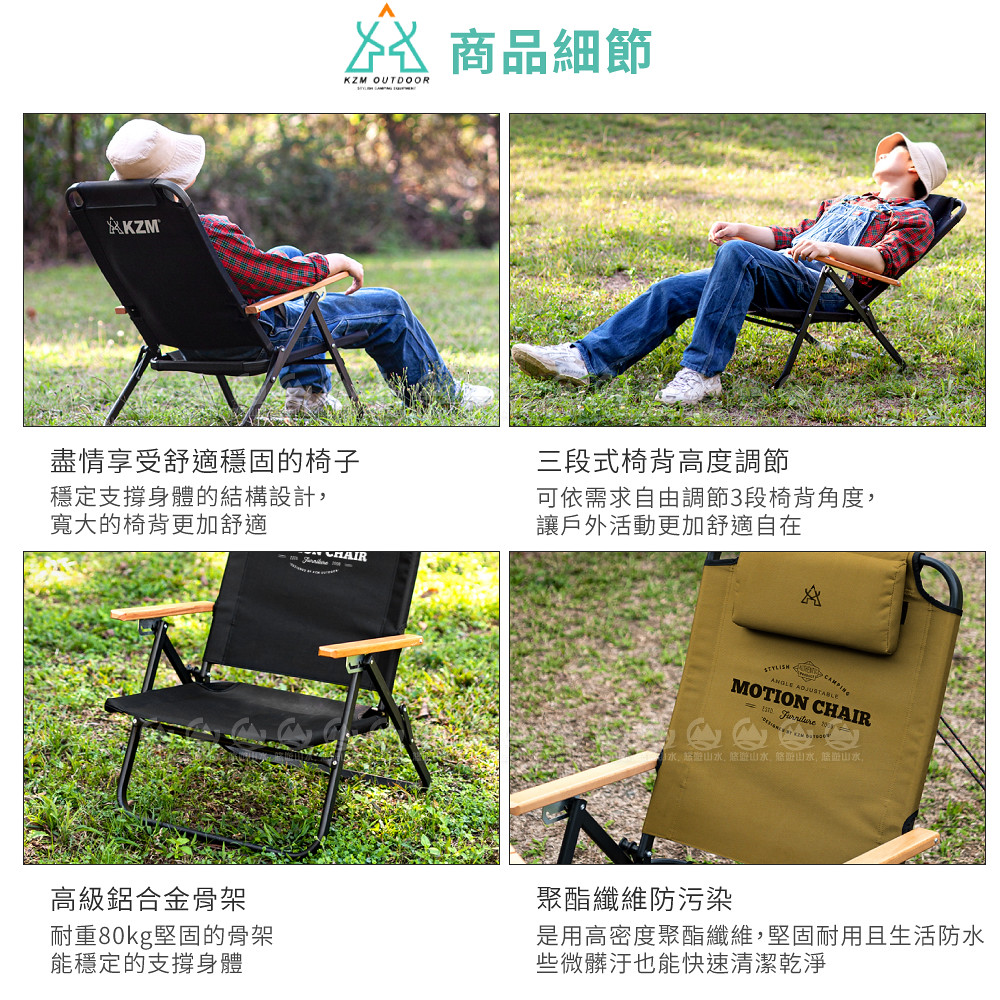The image is a grid layout of four pictures, presented on a plain white background. At the top center, in blue-green text, it features a logo with line outlines of two deer and an orange peak, accompanied by the label "KZM Outdoors" in black print. Below this are four Chinese characters in blue-green. 

The upper left picture shows the back of a metal and wooden fold-out chair with a black fabric seat, labeled "KZM" in white print. A person is lounging in the chair, seen from behind, wearing a floppy tan hat, blue overalls, and a red and black checkered flannel shirt with rolled-up sleeves. The upper right picture captures the same individual from the front, relaxing in the chair, looking off to the left side with arms resting on the wooden armrests. He is dressed in jeans and a checkered shirt, seated on grass under the sun. 

The lower left picture is a close-up of the empty black chair, showcasing its folding design, metal build, and wooden arms, set on a grass backdrop. The lower right picture depicts a similar chair but with a brown backrest, labeled "Stylish Camping Motion Chair Angle Adjustable" in black print, featuring a pillow at the top and dried grass in the background.

Each image is accompanied by black Chinese text beneath them, providing additional details. The chairs are described as canvas, slightly reclining with wooden arms, suitable for outdoor activities, likely promoting outdoor equipment in an advertisement format.